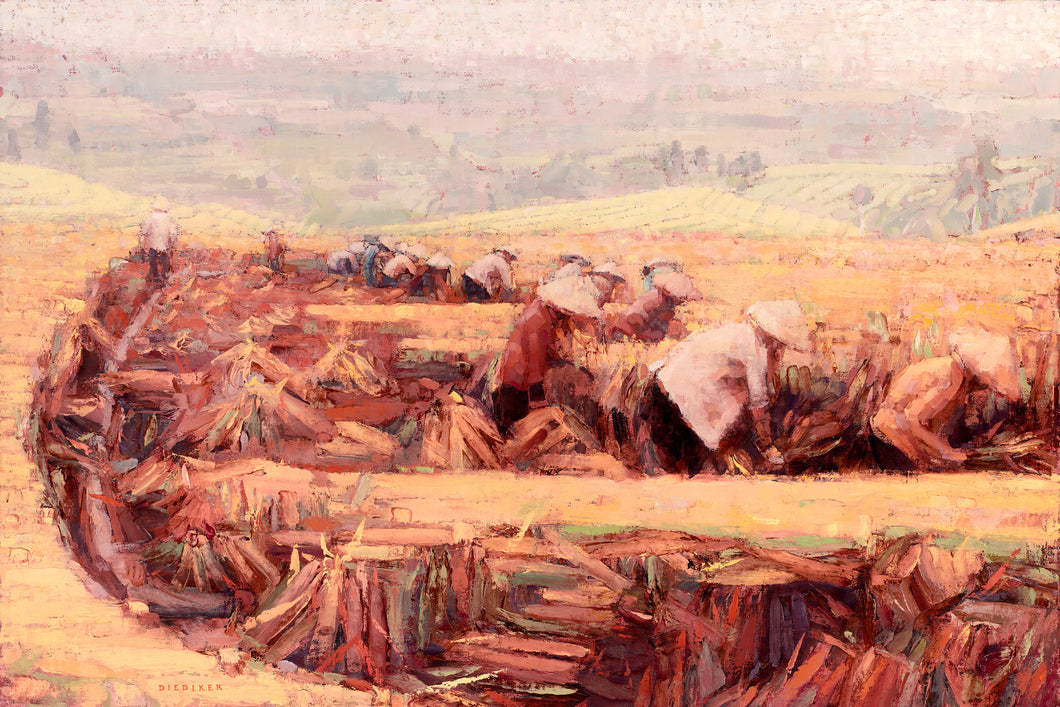This old painting depicts a vibrant scene set in a field, where a group of Asian women wearing straw sunhats are engrossed in their labor. They are standing in a row, bending over as they work diligently, possibly harvesting wheat or another crop. The intricate details reveal a variety of shapes and colors, contributing to the painting’s overall rich texture. Some women appear to be holding short-sized tools, possibly used for cutting down the wheat. Additionally, scattered around the field are objects that resemble corncobs, adding to the viewer’s curiosity about the setting. The background of the painting contrasts with the detailed foreground, featuring faint pastel colors, which give it an unfinished look. Despite this, the bottom portion is richly detailed, showcasing the artists’ emphasis on the labor and effort of the workers. The scene captures a snapshot of rural life, highlighting both the physical toil and the communal effort of the women in the field.